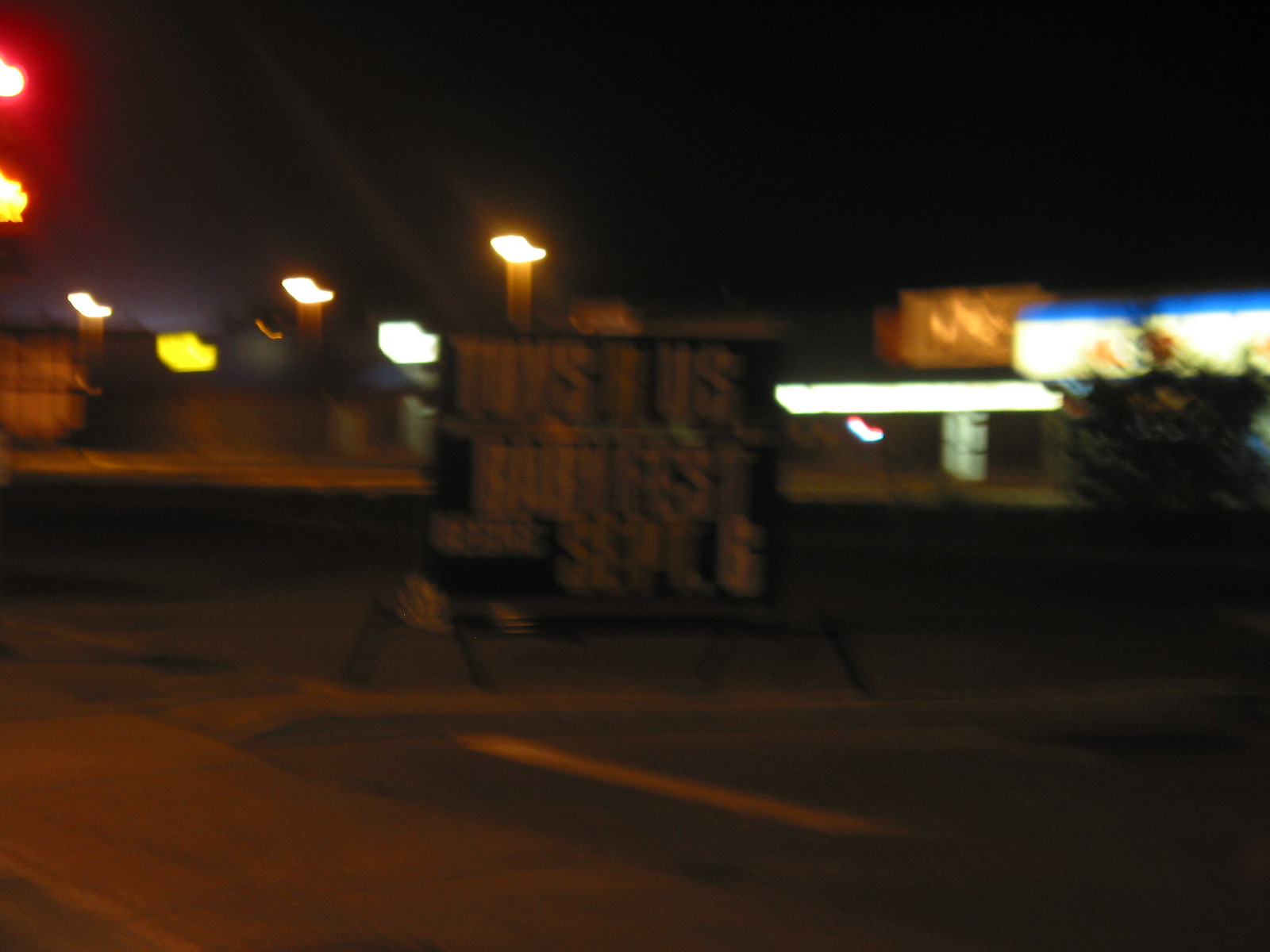The image depicts a very blurry night scene in a car parking lot, likely within a strip mall or commercial area in America. The centerpiece of the photo is an A-frame sign with white letters on a black background, though the text is largely illegible due to the blur. The sign seems to read something along the lines of "Toys R Us, Baby Fest" with a date, possibly September 6th. Surrounding the sign are various lights—parking lot lights, neon lights, and illuminated store signs—casting a glow against the dark, black sky. In the background, indistinct buildings are visible, along with faint shapes that might be trees or bushes, contributing to the overall obscurity of the scene. The image captures the essence of a commercial hub at night, characterized by its illuminated ambience and indistinct structures.